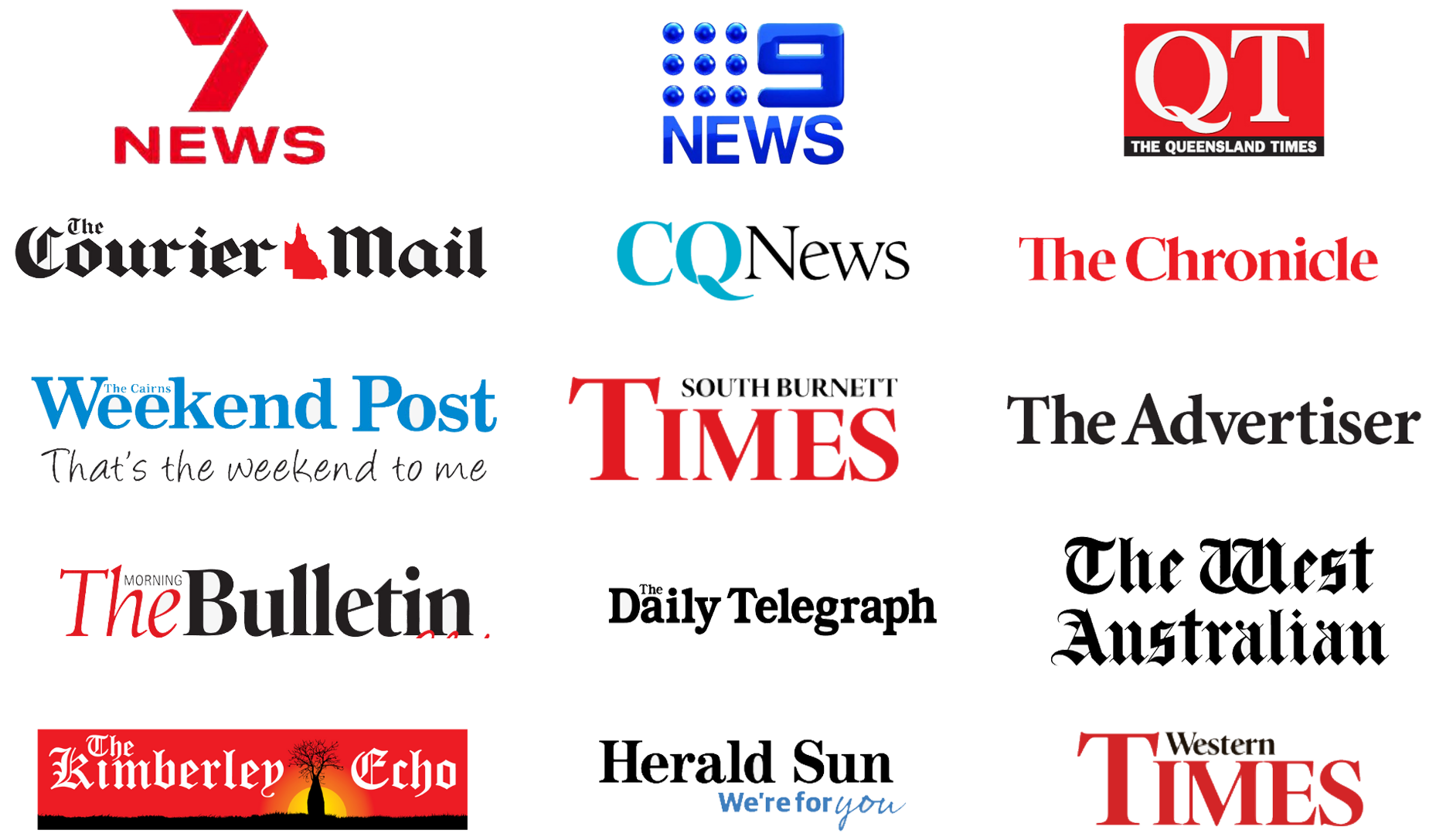This image is a screenshot set against a solid white background, showcasing three rows of various publication logos. 

**First row:**
- On the left, "7 News" is displayed prominently in red text, adhering to the distinct logo and style of the news network.
- Below it, "Courier Mail" appears in black text.
- Further down, the "Weekend Post" logo is presented in large blue text, accompanied by the phrase "That's the weekend to me." in black text.
- Following that, "The Bulletin" is listed, succeeded by "The Kimberley Echo".

**Second row:**
- At the upper right, the "9 News" logo is featured, with the number 9 in blue and smaller block text, accompanied by blue bullet points.
- Below, the "CQ News" logo is displayed.
- Next, "The South Burnett Times" is clearly labeled, with "Times" in prominent red block text.
- Following this, "The Daily Telegraph" appears in black text.
- Finally, "Herald Sun" is also listed in black text.

**Last row:**
- At the top, within a red box, the logo reads "QT" with the expanded name "The Queensland Times".
- This is followed by logos for "The Chronicle", "The Advertiser", "The West Australian", and lastly, "Western Times".